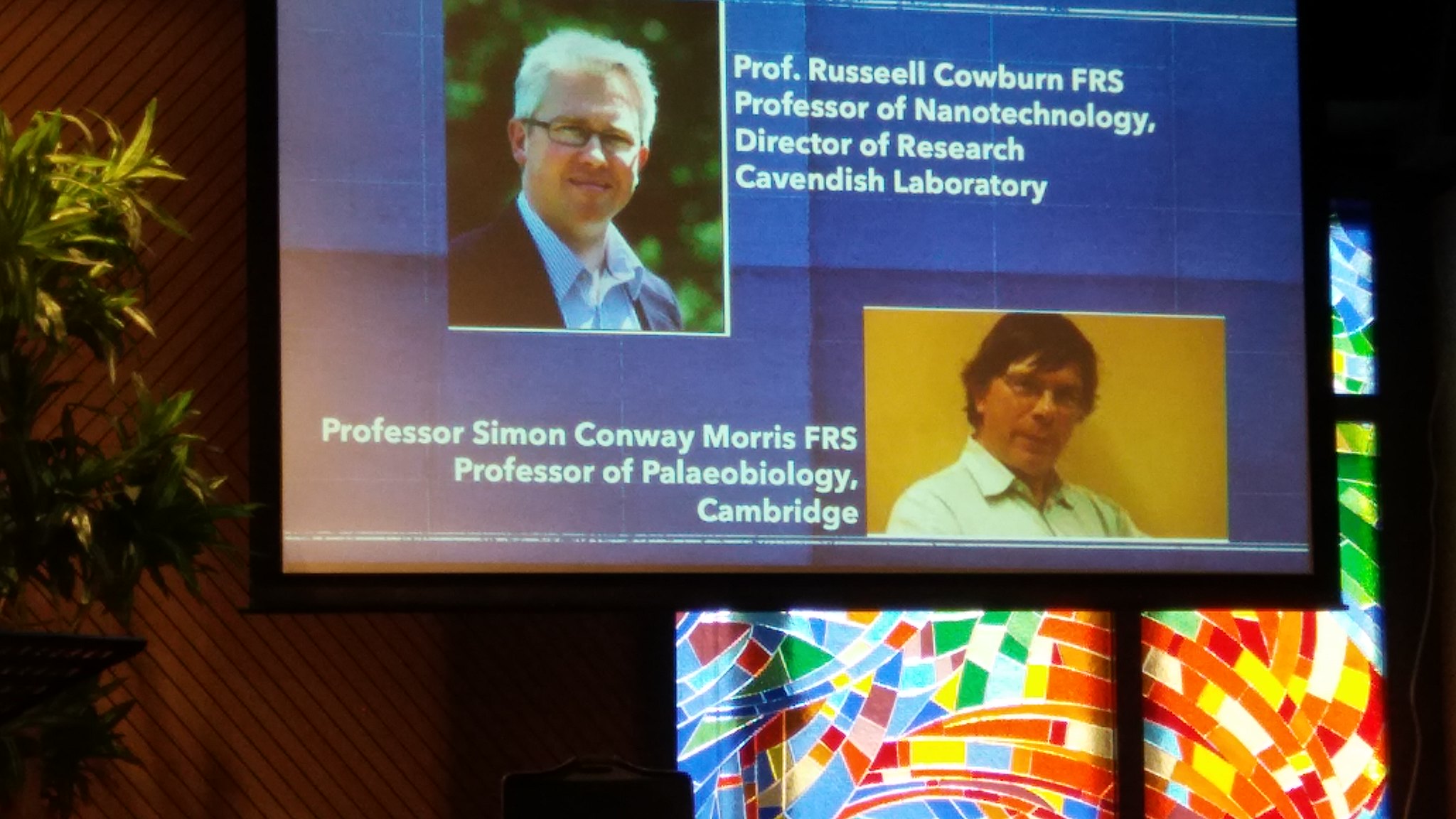The image displays a projected screen, likely from an overhead projector, featuring two prominent figures in academia. On the top left, there is a portrait of a white-haired man with glasses, identified by the white text to his right as Professor Russell Calburn, FRS, Professor of Nanotechnology and Director of Research at the Cavendish Laboratory. On the bottom right, there is another portrait of a dark-haired man with glasses, identified on the left side in white text as Professor Simon Morris, FRS, Professor of Paleobiology at Cambridge. The projection appears to be part of a slideshow, set against a blue background. The scene is on a stage, with a plant visible to the left of the screen and a multicolored, mosaic-like print in the background to the right.